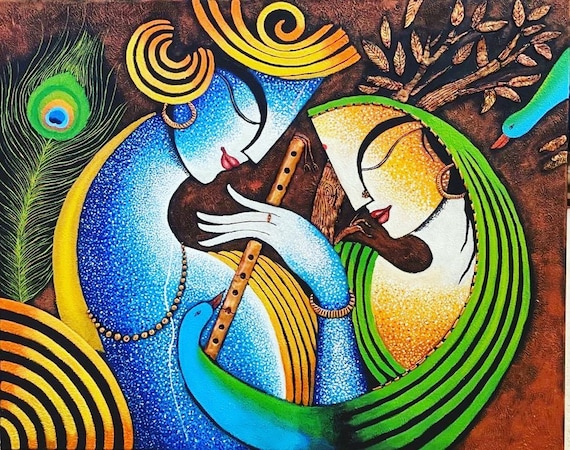In this intricate and colorful Doe La dance-inspired artwork, we see two central figures: a blue-skinned man and a green-haired woman. The man, adorned with golden hair, wears a gold necklace, a bracelet, and a ring on his hand, which also holds a flute. His forehead is vividly painted in color, and he too wears earrings. The woman, with her pink lips and fully closed eyes, is marked by red dots in her hair, which is a vibrant lime green. Her ears are adorned with earrings, and she also wears a golden copper bracelet and a ring on her hand.

The woman’s hair stretches out across the man's chest, transforming seamlessly into the head of a bird. This bird has a blue head and a brown beak. To the right, another bird's head is visible, painted green on the top and blue on the bottom with a similarly shaded beak. Nearby, to the far left of the image, there is a peacock tail, showcasing black and green colors. The surroundings are rich with intricate patterns, including a peacock-like leaf detail behind the woman and plant elements with brown leaves. The whole scene is set against a brown background, which further contrasts and highlights the colorful details present in the artwork. At the bottom left corner, circles radiate outward in black and golden or brown hues, adding to the mesmerizing visual complexity of the painting.